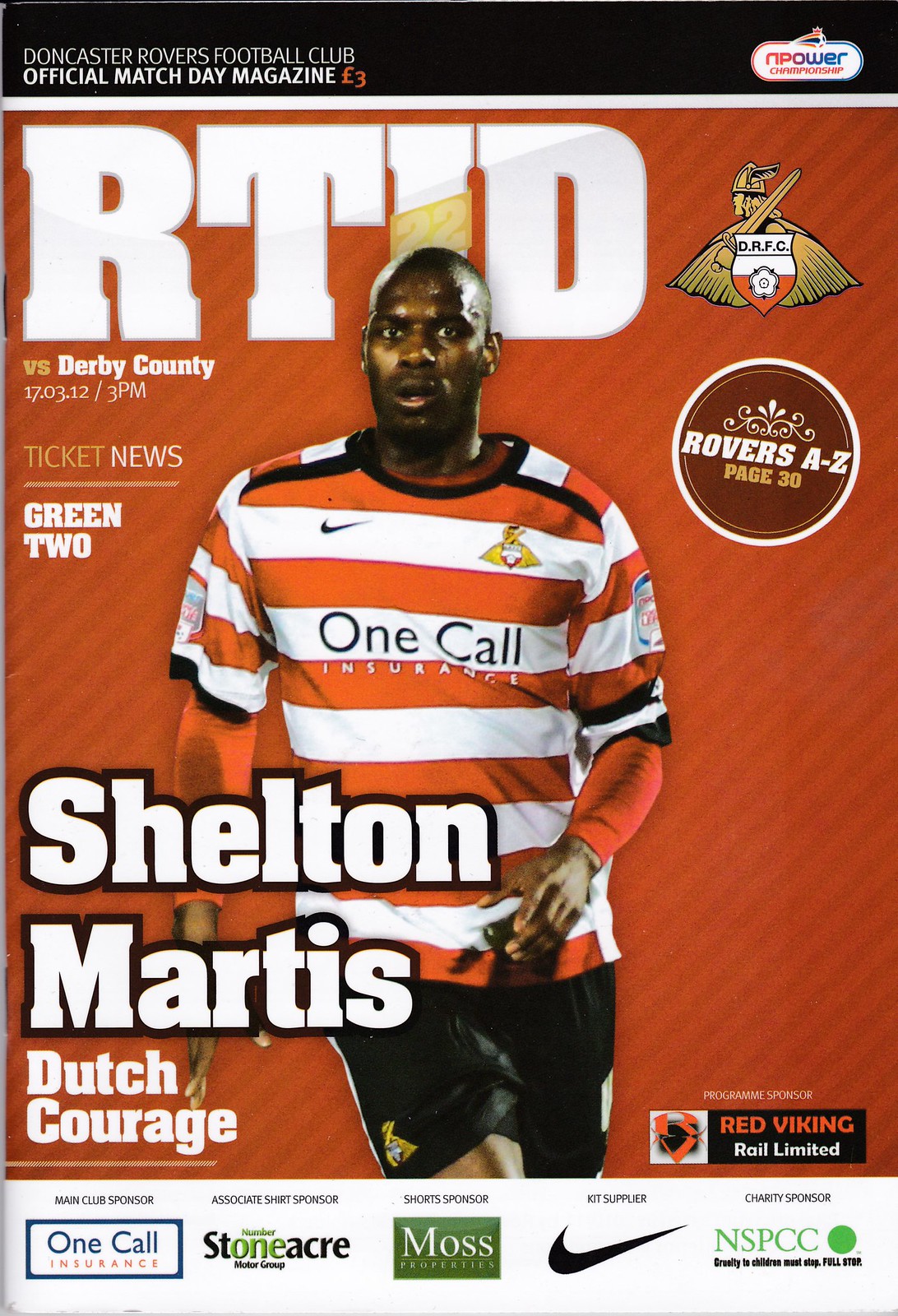The image features the front page of a Doncaster Rovers Football Club official match day magazine, promoting a match against Derby County, scheduled for 12-03-12 at 3 PM, priced at $3. At the top, it displays the club's logo, "Doncaster Rovers Football Club" in white letters on a black background, with "R-T-I-D" prominently underneath. 

Dominating the center is a photograph of Shelton Martis, an African-Dutch football player, wearing a red and white horizontally-striped jersey with "One Call" and other emblems on it, paired with dark blue shorts. His name "Shelton Martis" and the phrase "Dutch Courage" are inscribed in bold white letters below his image. Over his left shoulder, it reads "Rovers A to Z, page 30."

The magazine cover sports an orange background with white text in some areas and accents in black bold. Featured advertisements along the bottom include One Call Insurance, Stoneacre, Moss on a green background, the Nike Swoosh, and NSPCC in green on white. The layout and style, along with the attire and design elements, suggest this promotional material dates back a couple of decades.